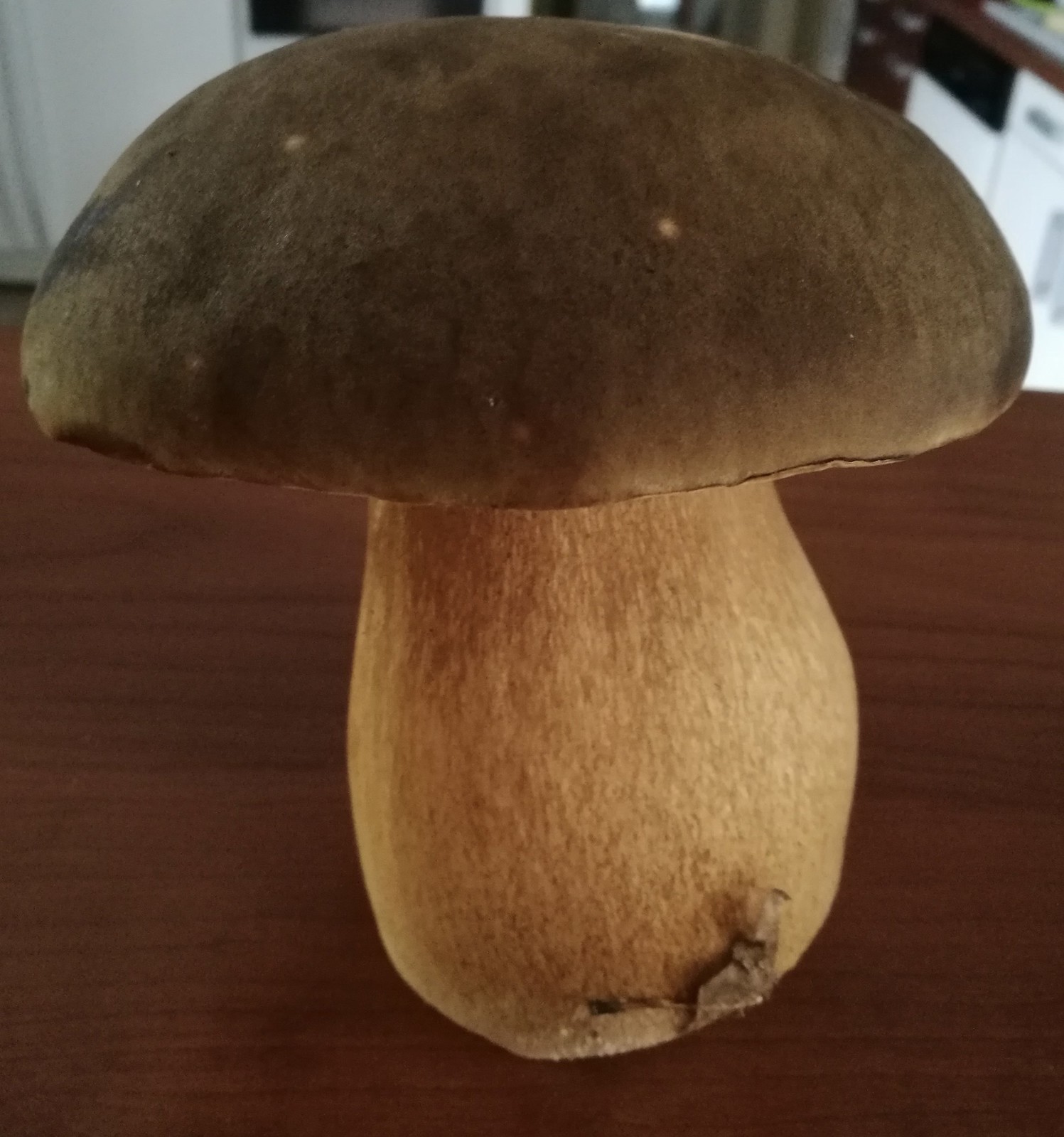The image showcases a prominent, large mushroom standing upright on a medium brown wooden desk or tabletop. The mushroom, which has a wide and thick stem, exhibits a light tan color with a textured surface. The domed cap of the mushroom is dark brown, peppered with smaller lighter-colored spots, and there seems to be a leaf stuck to the bottom of it. In the background, a kitchen setting is visible, featuring white lower cabinets with light gray trim and some black appliances. The countertop matches the medium brown wood of the desk. The intricately textured mushroom takes center stage in this indoor scene.